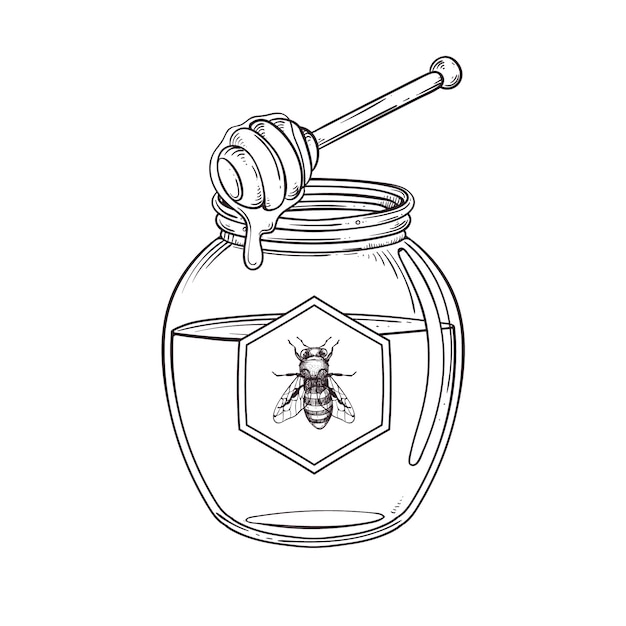This black-and-white sketch depicts a glass jar filled three-fourths with honey, set against a white background. The jar is short and wide, and prominently features a hexagon-shaped label with a bee. The bee's head is positioned at the top of the label, its wings pointing downward, and its tail at the bottom. Hovering above the jar is a honey dipper with fabric tied to one end, from which honey appears to be dripping onto the outside of the jar. The minimalistic style of the digital painting, characterized by deliberate brushstrokes, emphasizes the scene's simplicity and the key elements of the honey jar, the bee, and the honey dipper.